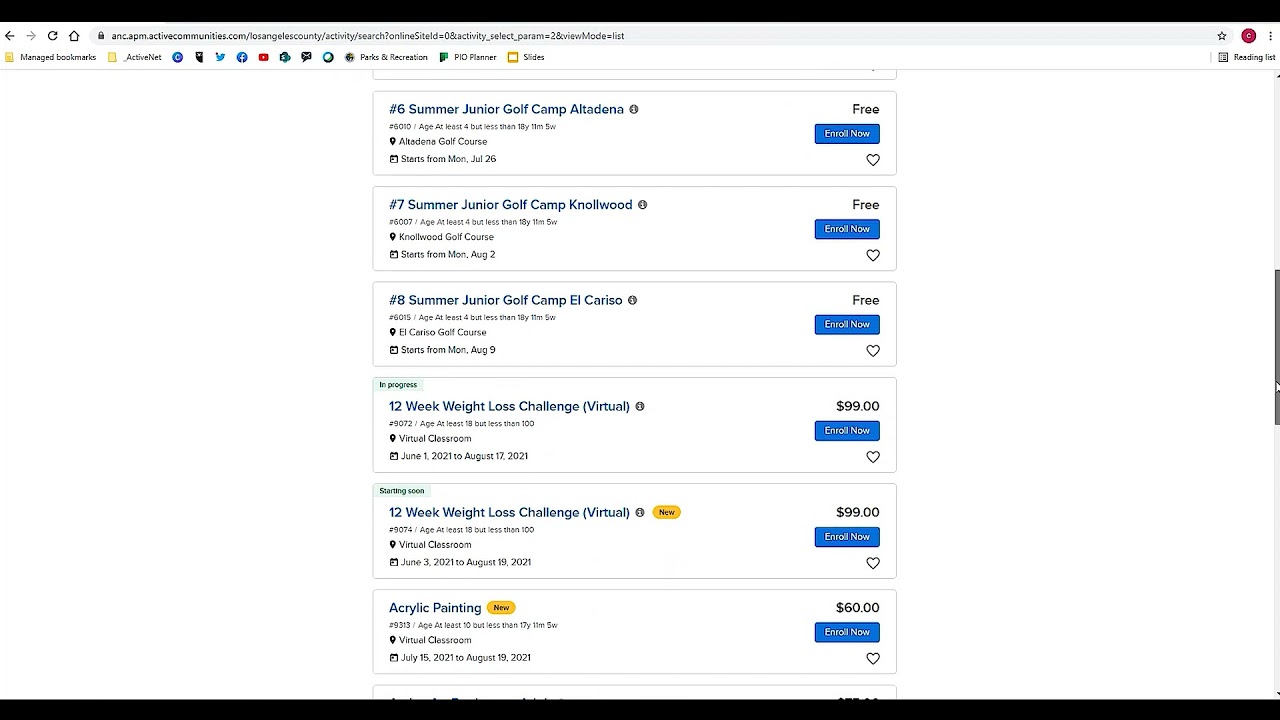**Screenshot Display of Los Angeles County Activities and Camps**

The screenshot showcases a variety of activities, classes, and camps available for enrollment in Los Angeles County, accessible via the URL: [anc.apm.activecommunities.com/LosAngelesCounty/activity/search?onlineSiteID=0&activity_select_param=2&viewMode=list](anc.apm.activecommunities.com/LosAngelesCounty/activity/search?onlineSiteID=0&activity_select_param=2&viewMode=list).

The listed activities in the screenshot include:
1. Summer Junior Golf Camp at Altadena (ID: 6)
2. Summer Junior Golf Camp at Knollwood (ID: 7)
3. Summer Junior Golf Camp at El Carrizo (ID: 8)
4. 12-Week Weight Loss Challenge (Virtual)
5. Acrylic Painting Class

Each entry provides the opportunity for participants to engage in a range of educational, recreational, and fitness activities, catering to various interests and age groups.